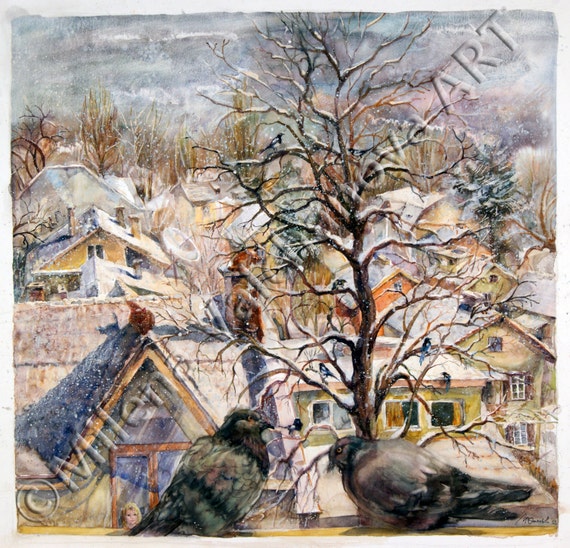The artwork, likely a drawing with textual watermark elements, features a wintery village scene dominated by a large, leafless tree at its center, dusted with snow. The rooftops of a cluster of similar looking houses, all blanketed in snow, stretch out behind the tree. A gray, overcast sky looms in the background, adding to the scene’s chilly atmosphere. Some trees in the background are bare while others, including pine trees, add touches of green despite being snow-covered. In the foreground, on a ledge at the base of the image, two plump pigeons—one with a grayish-blue hue and black head, the other more gray and black—face each other inward. At the bottom left corner, a partially obscured watermark with a circled C and the text "Milena Nova Art" can be seen faintly. The painting captures a quiet, dense village under a light snowfall, with fine details such as a white satellite dish on one of the homes and a blonde-haired girl peering through a window, accentuating the serene ambiance.